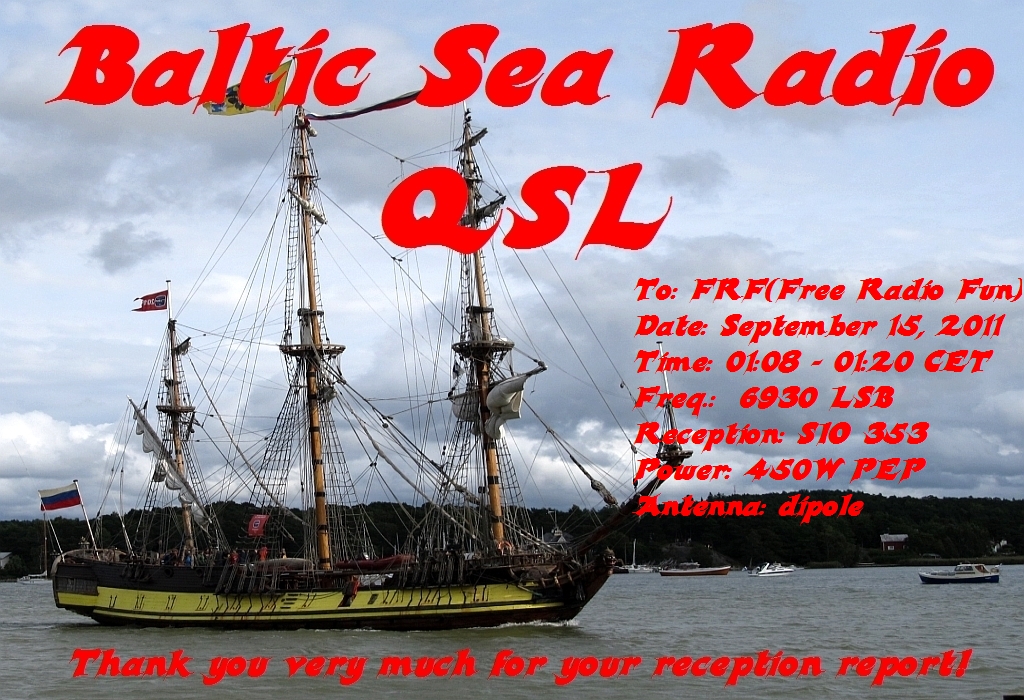This color photograph, taken outdoors on a cloudy day, features an old-timey, wooden sailing ship reminiscent of a pirate vessel, anchored in what appears to be a bay or lake. The ship, with its historic design, boasts a black hull adorned with a yellow stripe that spans across the bow. It has three yellow masts, each carrying different flags. Among these are a horizontally striped flag in white, blue, and red, a red flag with the letter 'G' on it, another red flag with different lettering flying overhead, and a yellow flag on the crow's nest, the text on which is illegible. Notably, none of the sails are hoisted. The image also includes a few modern-day boats in the water and dense trees in the background. Additionally, overlaid atop the image in red text is a detailed reception report that reads: "Baltic Sea Radio QSL-2FRM Free Radio Fund Date September 15, 2011 Time 01:08-01:20 CET Frequency 6930 LSB Reception Power 450W," followed by a thank you note for the reception report.